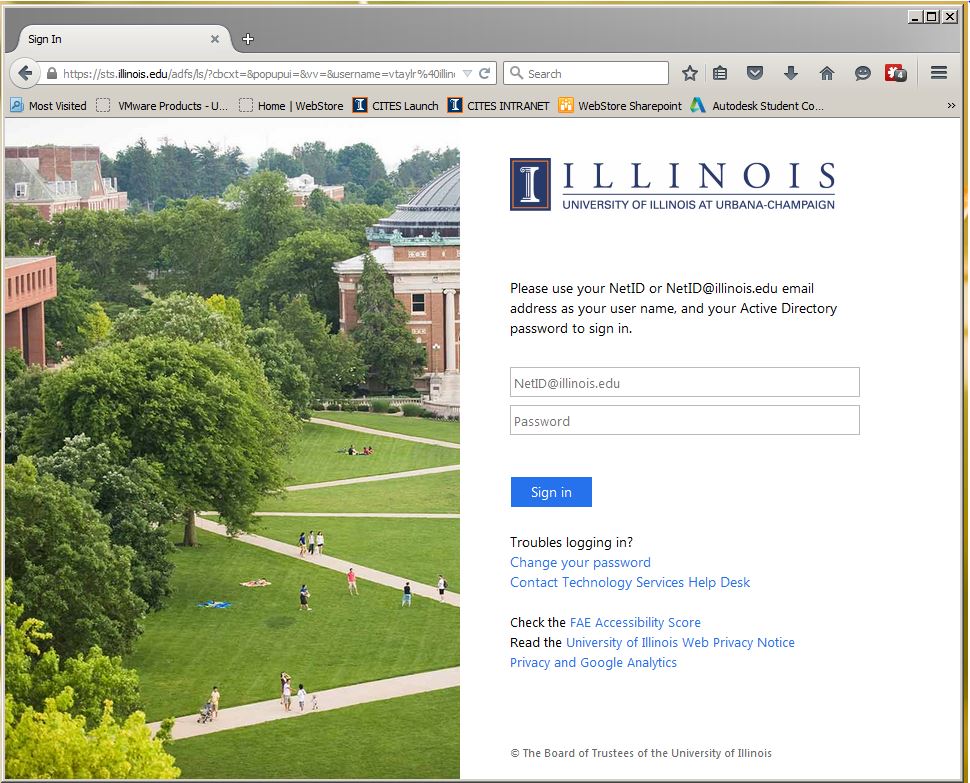A screen capture from an older computer, likely running Windows 95, is shown. The user interface is distinguishable by the characteristic layout and design of the minimize, maximize, and close buttons at the top right corner, along with a classic Windows 95 style ribbon. The main field of the image displays a webpage featuring a login page for the University of Illinois at Urbana-Champaign.

On the left half of the screen, there is an aerial photograph of the university commons area, showcasing trees on the left side and people walking around the grounds. On the right side of the image, the text prominently displays "University of Illinois at Urbana-Champaign." Below this, instructions are provided: "Please use your NetID or netid@illinois.edu email address as your username and your Active Directory password to sign in."

Two horizontal input fields are shown for the email and password, followed by a blue "Sign In" button. Additional options are listed beneath for troubleshooting such as "Trouble logging in?", "Change your password," "Contact Technical Service Help Desk," "Check the FAE accessibility score," and "Read the University of Illinois web privacy notice, privacy, and Google Analytics."

Overall, this is a detailed login page for the University of Illinois.